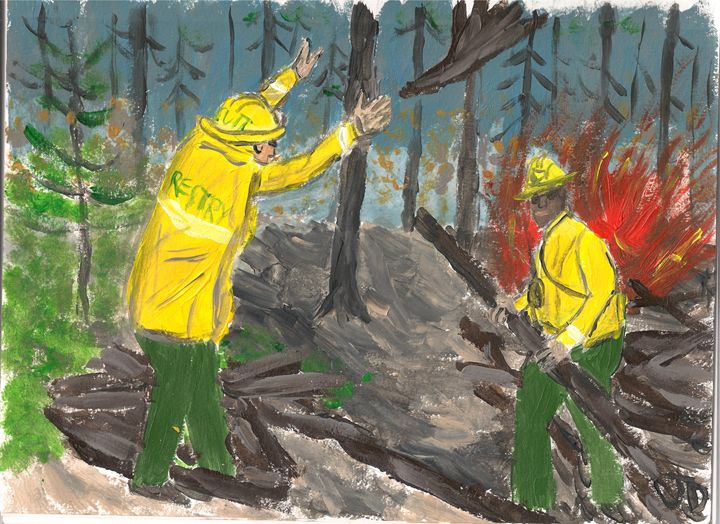The painting depicts a forest scene with two firefighters engaged in a controlled burn. The two men, distinguished by their yellow helmets, yellow jackets, and green pants, stand amidst tall, mostly barren trees with a bright red fire in the background. The Caucasian firefighter on the left, with "R-E-S-T-R-Y" inscribed on his jacket, stands with his arms raised, seemingly in a moment of surprise or disbelief, perhaps in response to the log the African American firefighter on the right is holding. This firefighter faces the artist directly, holding a tree log. The fire to the right is vivid, with red and yellow flames contrasting against the dark, grayish-blue sky and the bare, dark brown tree trunks. Some green leaves are still visible in the less affected parts of the forest. The overall scene is rendered in an abstract or naive art style, suggesting a somewhat simplistic and youthful interpretation of the intense moment.